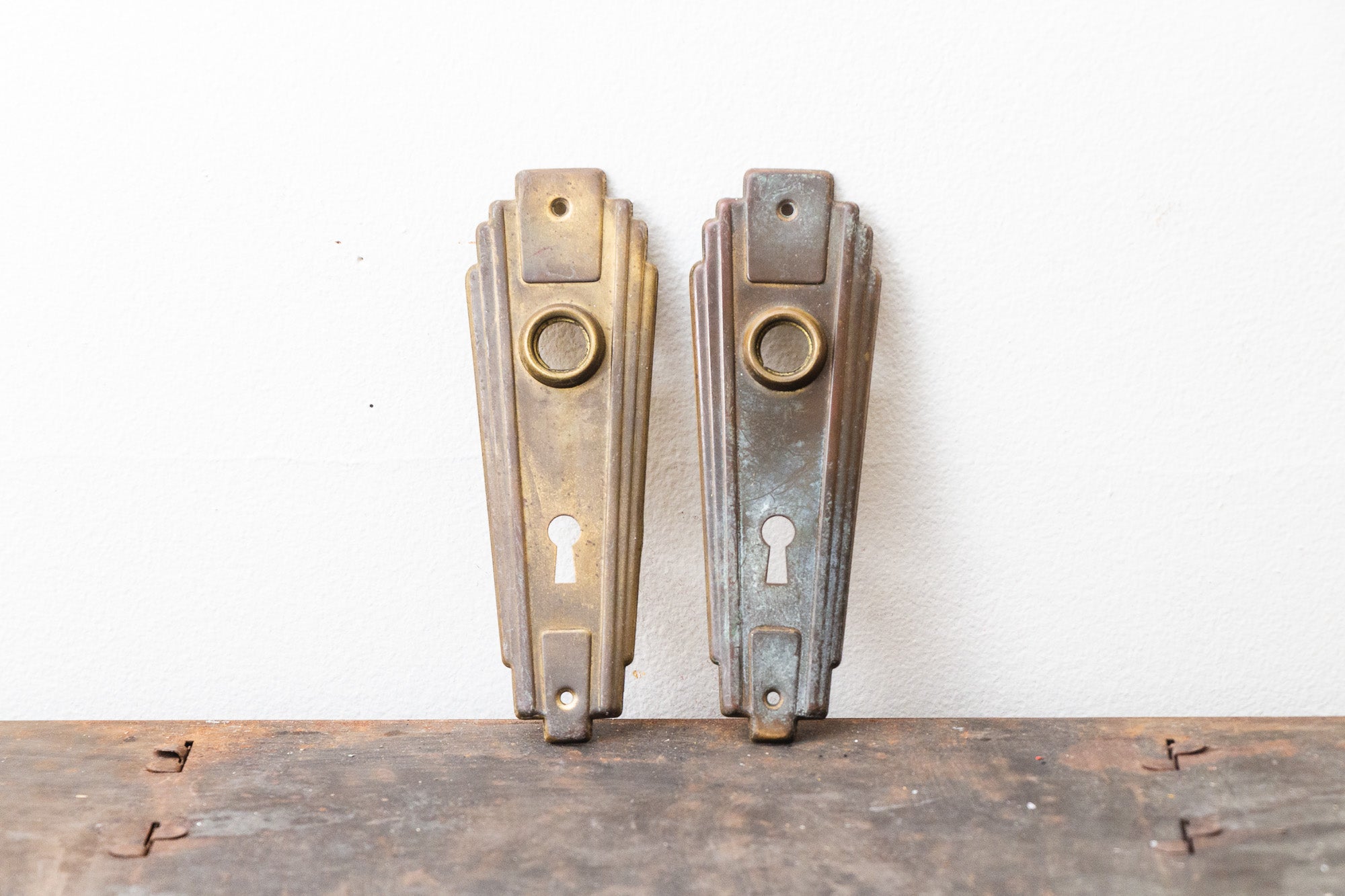This image showcases two antique metal keyhole covers designed in an art deco style, likely originating from the 1800s or 1900s. Each faceplate features a circular top with an oblong square bottom, indicative of old-fashioned craftsmanship. Both keyhole covers are similar in shape, size, and decorative elements. The cover on the left gleams with a brighter gold finish, suggesting it has been polished, while the one on the right displays a darker, distressed bronze hue. They are positioned against a white wall and rest on a weathered wooden surface resembling a chest or shelf, characterized by its rough texture and varying shades of brown and tan. The scene evokes a sense of historical elegance, with the aged wood possibly dusted from a recent sanding project.